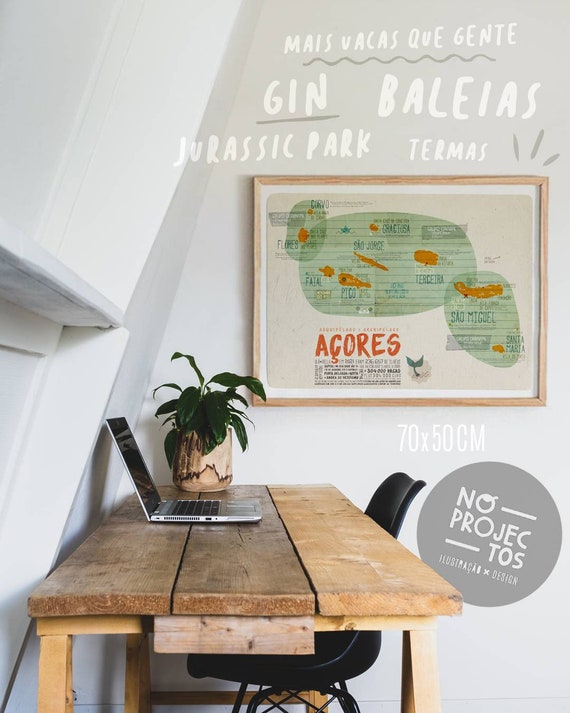This photograph captures a cozy, rustic home office setup nestled in what appears to be an attic with sloped white walls. The centerpiece is a desk fashioned from three sturdy wooden planks, supported by raw, unstained wooden legs. A sleek silver laptop with a black keyboard sits on the desk next to a tan and brown flower pot with a thriving green plant. Below the desk, a small black plastic chair is positioned neatly. On the whitewashed wall, there's a rectangular framed artwork. The artwork features a map-like illustration of islands, with green geometric figures, and bears the inscriptions “Jan Ballez, Jurassic Park, Termas” and “70 by 50 centimeters.” Additionally, some words in Spanish, including “Nos Projectos,” are visible. Cabinets align the left side of the space, and overall, the scene exudes a warm, makeshift workspace vibe.